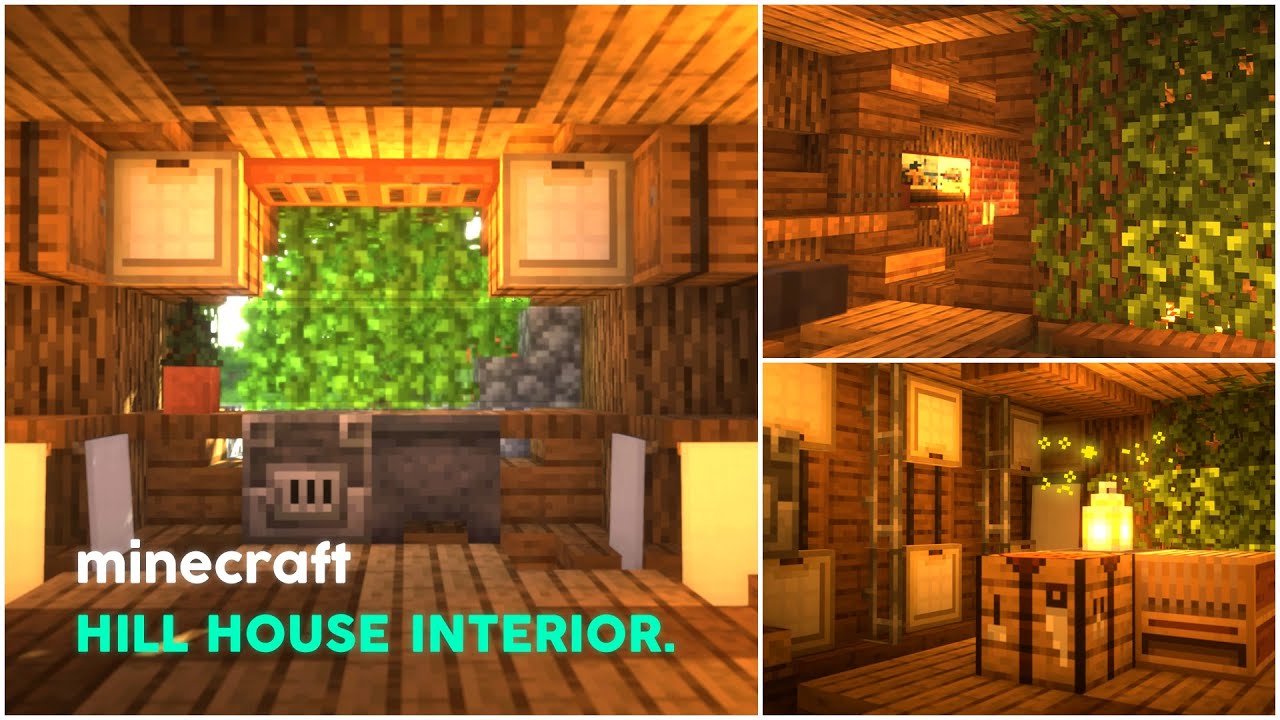The image is a detailed collage depicting a beautifully crafted interior of a "Minecraft Hill House," clearly labeled as such with "Minecraft" in white lowercase letters and "HILL HOUSE INTERIOR" in turquoise uppercase letters. The collage consists of three sections: one large square image to the left and two smaller, rectangular images stacked on the right. 

The main large image on the left showcases a cozy kitchen area within the Minecraft house, featuring a blend of various wood types including dark and light woods. Noteworthy elements include a window with a view of greenery outside, a cauldron, a furnace, a wooden workbench, and barrels. The ceilings are adorned with trapdoors used creatively to form a window. The warm and inviting lighting, enhanced by a mod, adds to the atmosphere, casting a golden glow across the interior.

The top smaller image on the right displays a room with an artful fireplace and some wall decor, possibly artworks or frames, alongside moss or moss-like elements. This room continues the wooden theme and adds a sense of rustic charm and warmth.

The bottom smaller image on the right portrays another room featuring more wooden elements, a glowing lantern providing soft ambient light, a light brown ladder, and leafy green curtains that hang from the ceiling to the floor, contributing to the organic, nature-inspired decor.

Overall, the collage captures the essence of a thoughtfully designed Minecraft interior, with detailed touches and warm lighting that create a welcoming and homely atmosphere.